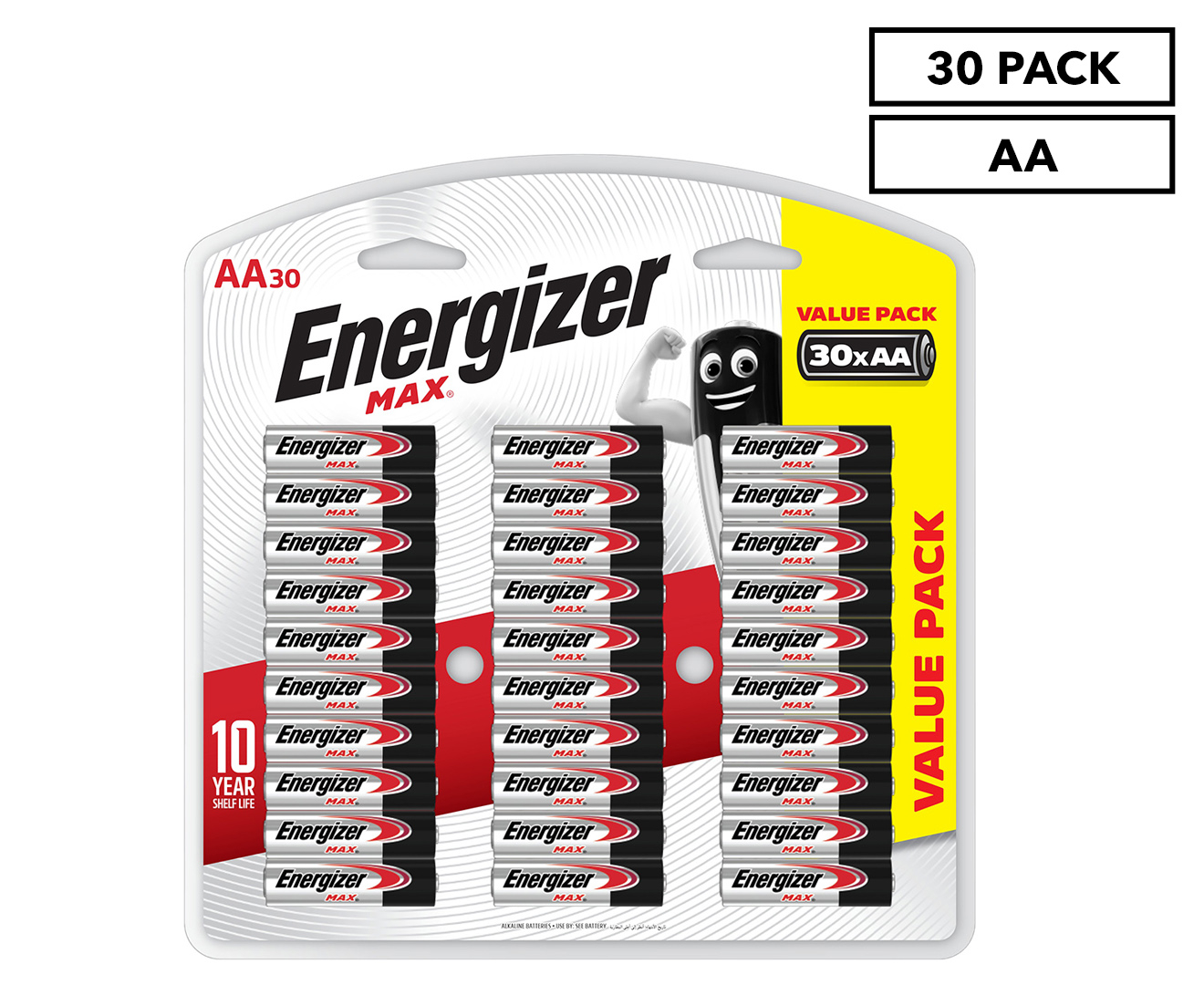This image features a packet of the ever-popular Energizer brand AA batteries. The plastic packaging is distinct, with square edges on the left, right, and bottom, while the top is rounded. It includes two holes, one on each side near the top, for convenient hanging on a store rack. The exterior of the plastic case is white.

In the upper left corner, "AA30" is written in red, indicating that there are 30 AA batteries in this packet. The main branding includes "Energizer" in black and "Max" in red, prominently displayed. A red label across the center proclaims a "10-year shelf life." On the right side, a bright yellow label reads "Value Pack," emphasizing the bulk purchase.

The batteries are arranged in three rows of ten, totaling 30 batteries. Each battery is silver with black and red text, featuring a red logo. The tops of the batteries are black. Additionally, one of the batteries in the background image is depicted with a flexing muscle and a character face, adding a touch of personality to the branding. In the upper right corner, "30-pack AA" is noted, confirming the quantity once again.